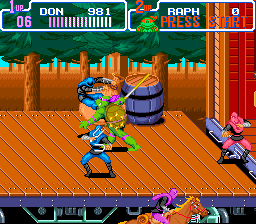In this vibrant video game scene, several dynamic characters are poised for action. At the forefront, a blue-clad warrior wields a gleaming sword, preparing to strike. Behind him stands a green turtle-like character, distinguishable by his green limbs, protective shell, and his own sword, adding to the tension. Above them, a blue-armored figure with visible arms and head appears to leap down into the fray, highlighting the scene's intensity. To the far right, a pink warrior with grey limbs stands ready, weapon in hand and prepared for combat. Adding to the rich tapestry of the scene, a purple wine barrel with black belts sits prominently. Below the stage, a horse gallops past rapidly, while the background is filled with a dense forest of identical trees, each with a brown trunk and lush green foliage on top. The setting atop the platform, akin to a truck bed, lends a unique sense of height and movement to the dynamic tableau.